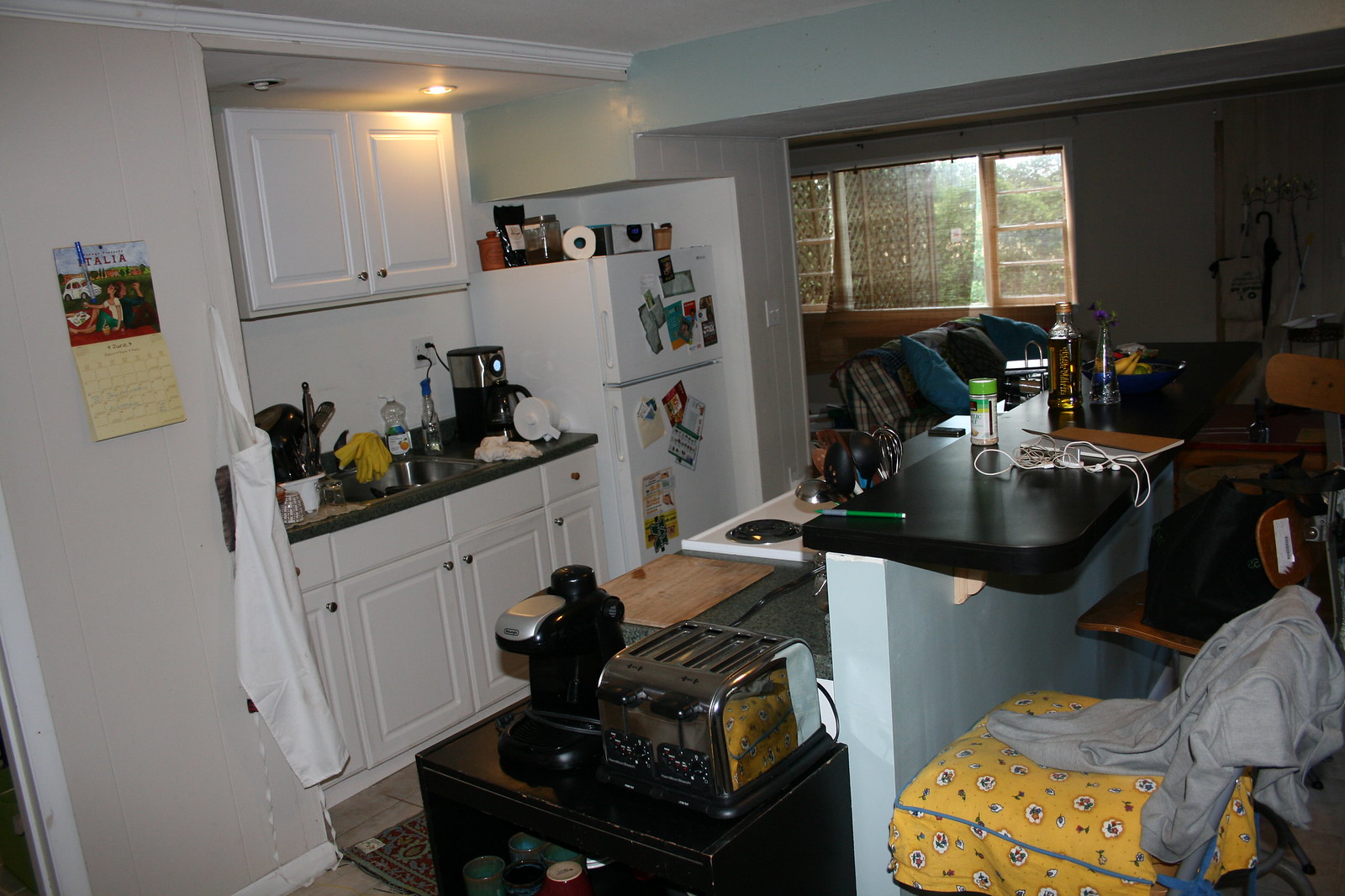The image is a color photograph showcasing the interior of a house, specifically focusing on the kitchen with a glimpse into an adjacent living area. The kitchen is compact and features a row of white wall cabinets and matching base cabinets. A dark-colored countertop spans across the cabinetry, culminating in a stainless steel sink. A partial wall to the left, cropped in the image, hosts a calendar and a nail with a hanging apron. This wall is light-colored and hints at a possible doorway beyond it. The area appears neat and functional, capturing the essence of a cozy domestic space.